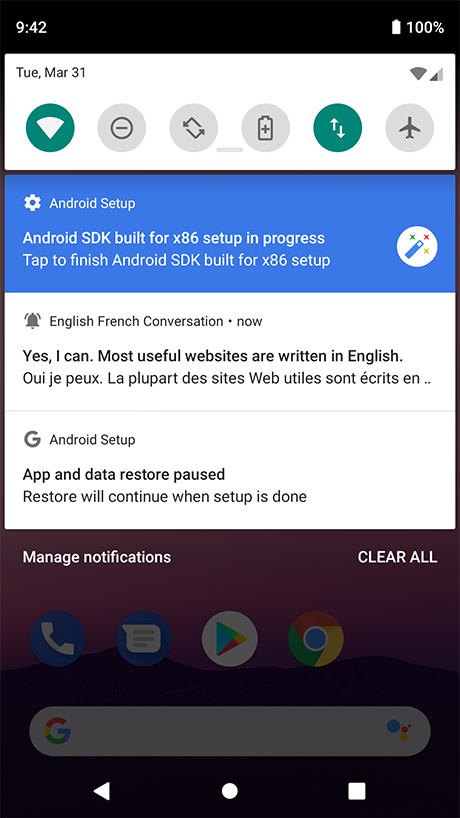The image portrays a screenshot from an Android device. At the top, a black status bar displays the time "9:42," followed by a full battery icon and a date reading "March 31." Nearby, it shows the Wi-Fi signal and mobile network strength symbols. 

Continuing down, there's a row of circular icons in various colors:
- A teal circle with a white Wi-Fi symbol.
- A gray circle with a black circle and a slash through it.
- A gray circle featuring two black arrows pointing in opposite directions.
- A gray circle containing a battery icon with a plus sign.
- Another teal circle displaying white arrows.
- A gray circle with an airplane icon.

Below this row, a set of blue boxes contains a white cogwheel, accompanied by text reading: "Android setup, Android SDK built for x86 setup in progress. Tap to finish Android SDK built for x86 setup." Adjacent to this text is a white circle with a blue magician's wand surrounded by teal, red, and gold stars.

Following this, two white boxes with black text appear:
- The first shows a bell icon next to the sentence "English, French conversation now. Yes, I can. Most useful websites are written in English," followed by French text "Oui, J-Po" and another French sentence.
- The second reads: "G Android setup, app and data restore paused. Restore will continue when setup is done." Below this, text reads "Manage notifications" and "Clear all."

Towards the bottom are various app icons:
- A blue and white phone icon.
- A blue and white text message bubble.
- A multi-colored icon for the Google Play Store (pink, gold, white, and blue).
- A Chrome browser icon (red, blue, gold, and green).

At the very bottom, there's a search bar featuring the Google icon with its characteristic red, gold, blue, and green dots. Directly below this toolbar, there are three navigation icons: a white back arrow, a white circle for the home button, and a white square for the recent apps.